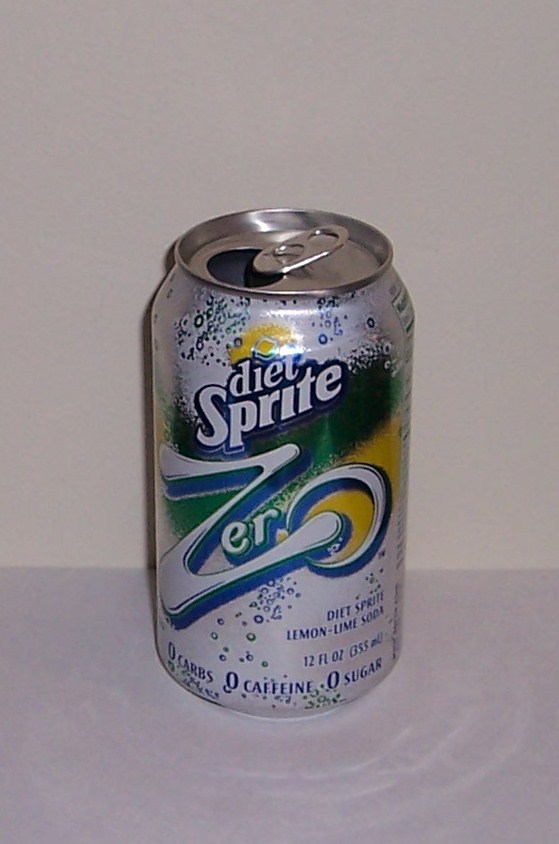This is a detailed color photo of an open can of Diet Sprite Zero. The can predominantly features a metallic white background with blue bubbles, complemented by traditional Sprite colors: vibrant green and bright yellow accents and blue outlines around the white text. The front displays the text "Diet Sprite Zero" with a stylized "ZERO" where the Z is larger than the other letters, followed by the description "Lemon Lime Soda." The bottom part of the can prominently states "Zero Carbs, Zero Caffeine, Zero Sugar." Measuring 12 fluid ounces (355 milliliters), the can is the sole focus of the image, resting on a light gray surface with a white beige wall behind it. This minimalist setting ensures that the attention is entirely on the can's design and its details.